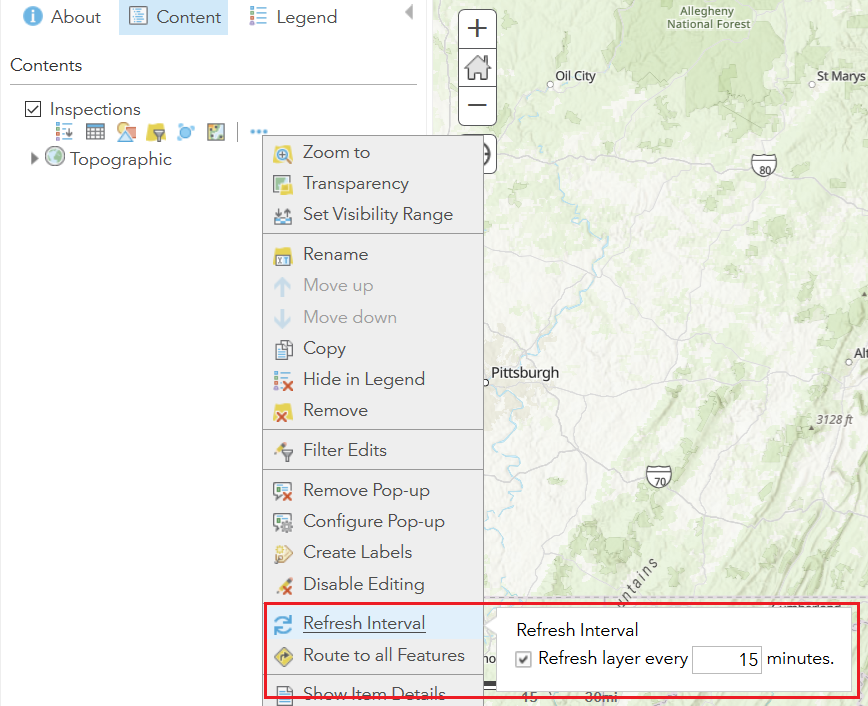The image features a split-screen composition. On the left side is a whiteboard background. At the top of this background, the text reads "About Content Legend." Near the bottom, the heading "Contents" appears, underlined by a horizontal line. Below this line, the word "Inspections" is displayed with a checked box beside it. Underneath, there are several unidentifiable icons, followed by an icon of the world labeled "Topographic." 

A menu is open beneath this, listing several options: "Zoom To," "Transparency," "Visibility Range," "Rename," "Move Up," "Move Down," "Copy," "Hide in Legend," "Remove," "Filter Edit," "Remove Pop-up," "Configure Pop-up," "Create Labels," "Disable Editing," "Refresh in Interval," and "Route to All Features." Each menu item is accompanied by an icon on its left.

The right side of the image shows a detailed map of an area near Pittsburgh, highlighting the Allegheny National Forest. The map includes various roads and small towns, providing a geographical context to the content displayed on the left side.